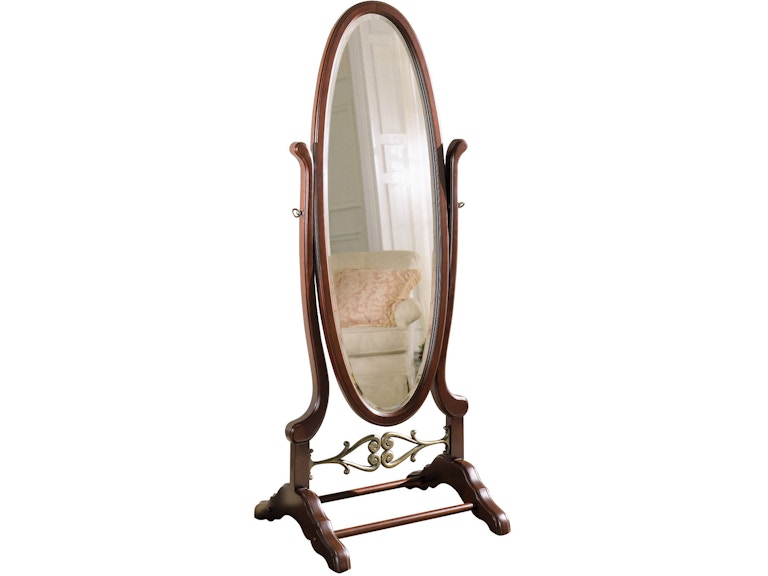This photograph features a vintage Victorian-style, full-length oval swivel mirror set against a completely white, cropped-out background. The mirror is framed in dark chestnut wood and attached to a freestanding wooden base with two legs that extend into four feet for stability. Between the two legs are supporting rods, including a decorative piece at the middle layer of the base that resembles a heart shape. In the reflection of the mirror, one can observe a living room with white walls or doors, a beige or white chair or sofa adorned with an orange or peach-colored pillow.